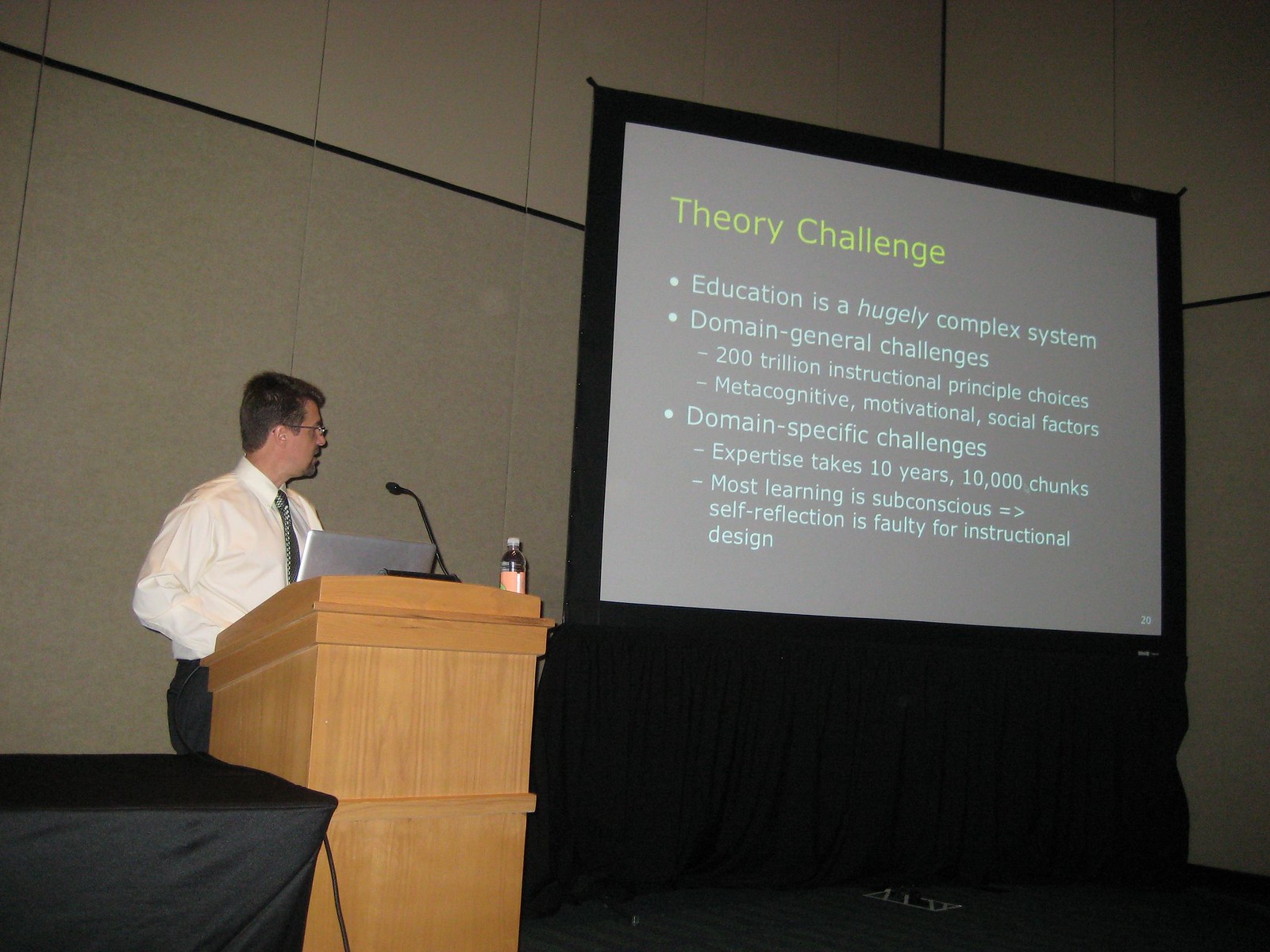In the image, a man stands behind a light brown wooden podium, which is adorned with a small black microphone and a gray Dell laptop. Atop the podium, there is also a bottle with an orange label and a plastic cap, possibly containing some beverage. The man, a white male with short dark hair, is wearing eyeglasses, a white long-sleeve button-down collared shirt, a dark tie, and black pants. He sports a goatee and stands with a composed posture. To his right, a projection board screen displays a PowerPoint slide titled "Theory Challenge" in yellow at the top. The slide contains three detailed bullet points: "Education is a hugely complex system," "Domain General Challenges" with subpoints "200 Trillion Instructional Principle Choices, Metacognitive Motivational Social Factors," and "Domain Specific Challenges" with subpoints "Expertise Takes 10 Years, 10,000 Chunks, Most Learning is Subconscious, Self-Reflection is Faulty for Instructional Design." To the left of the podium, there is a table covered with a black cloth. The man appears to be presenting or delivering a speech, looking slightly to his left at the projection.